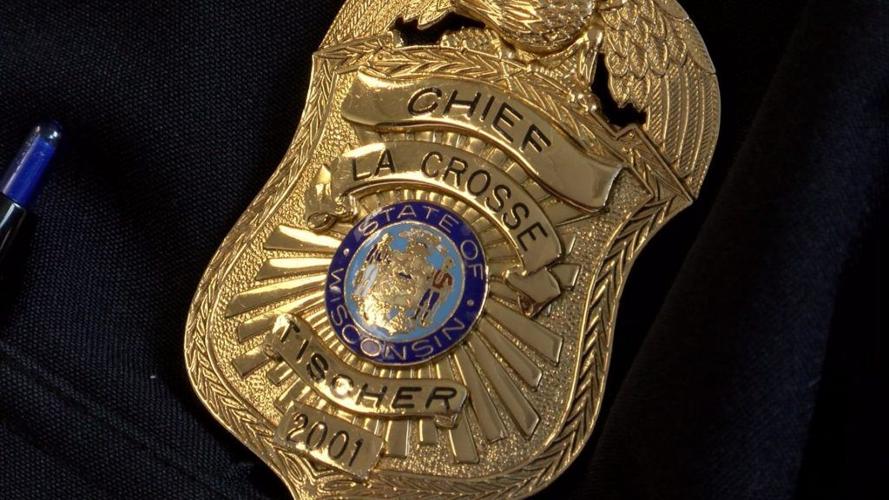This is a detailed, close-up photograph showcasing the breast pocket area of a dark navy blue police officer's uniform. The primary focus is a vibrant gold police badge. The intricate badge, featuring an eagle with wings spread at the top, contains several distinct sections with black lettering. At the top, 'Chief' is prominently displayed, followed by an arched sash reading 'La Crosse'. Below this, a circular emblem with gold lettering encircles a light blue center, detailing 'State of Wisconsin' and featuring the state's emblem. Underneath the circle, the name 'Tissier' is inscribed, accompanied by the number '2001' on a separate rectangular portion. Additionally, a blue pen is visible, protruding from the pocket on the left side of the image, enhancing the formal, utilitarian aspect of the uniform. The badge is pinned to the fabric, which has a noticeable cloth texture, suggesting it remains attached to the uniform. The arrangement, though slightly skewed to the right, remains meticulously detailed, highlighting the officer's rank and affiliation.